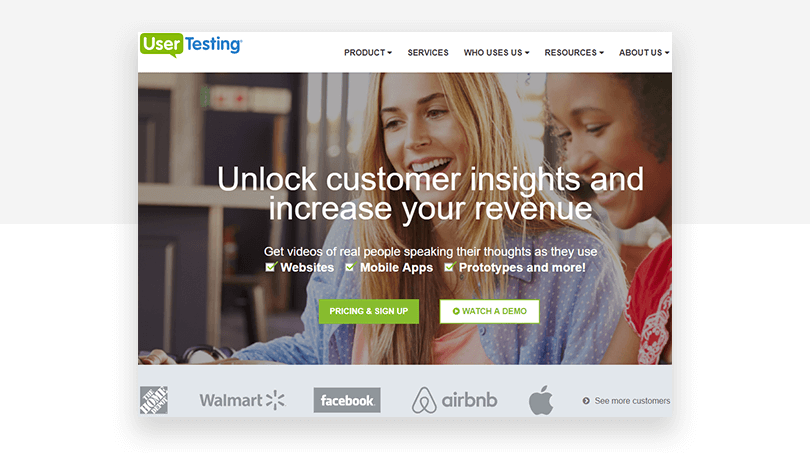This image is a promotional splash screen for the company User Testing.

At the center of the image, prominently displayed, is a large, slightly grayed-out photo of two women smiling—one with her mouth open in joy. This subdued visual effect highlights the accompanying text.

At the top of the image, there's a white banner. On the left side of this banner, "User Testing" is displayed, with "User" written in a white font set against a green, speech bubble-like background, and "Testing" in a larger blue font. On the right side of the banner are several navigation options in black font: Product, Services, Who Uses Us, Resources, and About Us.

The main message, in bold white font, is centered on the image and reads, "Unlock Customer Insights and Increase Your Revenue." Below this, in slightly smaller white font, it states, "Get Videos of Real People Speaking Their Thoughts As They Use." Beneath this text, green checkmarks highlight key features like "Websites," "Mobile Apps," "Prototypes, and More!"

At the bottom of the image, a gray banner displays logos of several prominent companies from left to right: The Home Depot, Walmart, Facebook, Airbnb, and Apple. To the right of these logos, the text "See More Customers" is displayed.

In the lower portion of the image, two call-to-action buttons are prominently placed. On the left, a green rectangle with white font reads "Pricing and Sign Up." To its right, a white rectangle outlined in green with green text reads "Watch a Demo," accompanied by a play icon.

This cohesive and detailed design effectively communicates User Testing's services and encourages user engagement through clear and appealing visual elements.